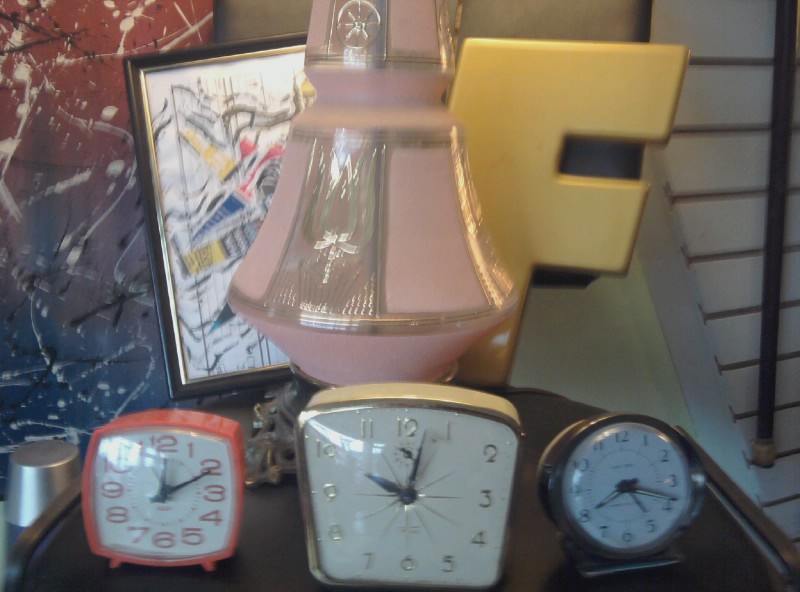A blurry photograph captures a vintage brown table in a thrift shop, adorned with eclectic items. Dominating the table's surface is the ornate base of a pink and gold lamp, exuding an antique charm. Beside it, three distinct, dated alarm clocks vie for attention; two with squarish designs and one, a classic round model, each displaying a different time. The backdrop features an array of propped objects—a squiggly abstract painting, another unusual framed artwork, and an eye-catching large plastic letter 'F' in bright yellow. A white wall behind these items holds what appears to be a walk-in cane, adding to the scene’s nostalgic intrigue.